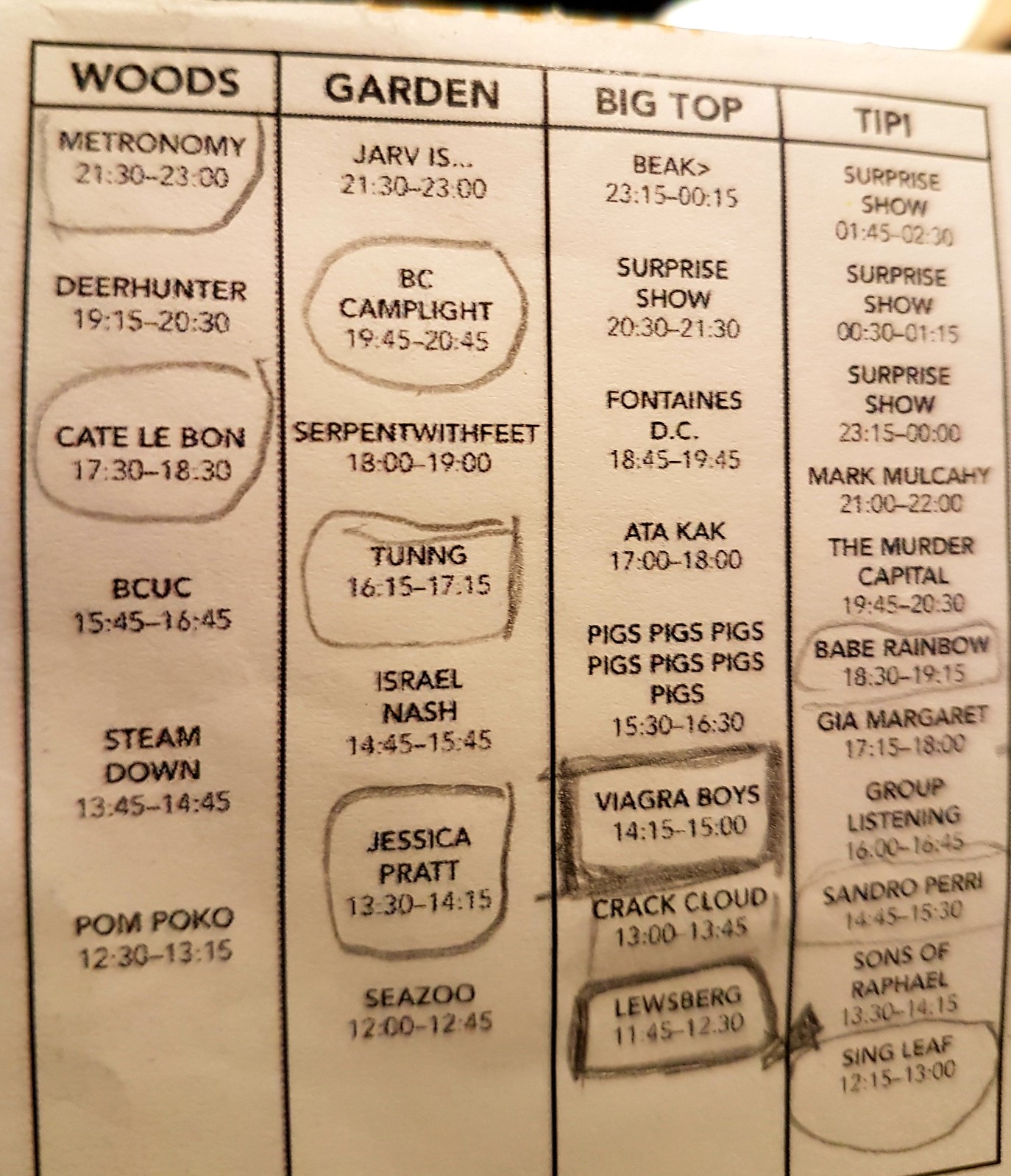The image depicts a slightly tilted sheet of brown paper, divided into four columns with solid black lines. Each column is headed by bold, capitalized text reading: "WOODS," "GARDEN," "BIG TOP," and "TIPI." Below these headers are listed various events, performances, or meetings with corresponding times. 

For example, under "Woods," six events are listed, including performances by Metronomy from 21:30-23:00, Deer Hunter from 19:50-20:30, and Cate Le Bon from 17:30-18:30. The "Garden" column lists seven events, while the "Big Top" has eight and "TIPI" boasts eleven, including the first four slots marked as "Surprise Show."

Some events are circled or boxed, indicating selections or preferences. Notably, the event "Viagra Boys" from 14:15-15:00 in the "Garden" column and "Luesburg" towards the bottom are heavily outlined with a pencil, drawing special attention. The right side of the image, and specifically the "TIPI" column, appears slightly blurred and out of focus.